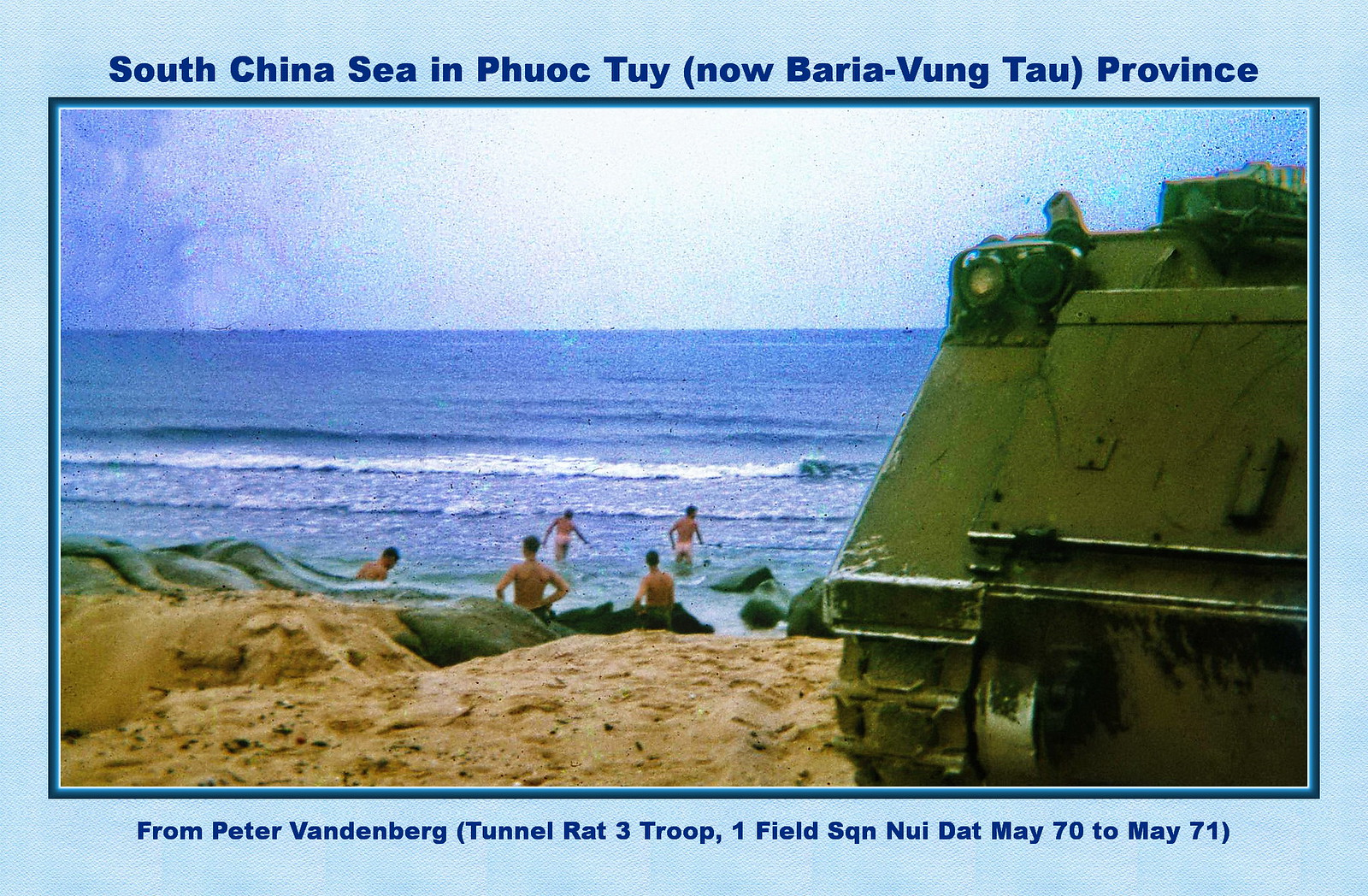This rectangular photograph, bordered by a light baby blue frame with dark blue text at the top reading "South China Sea in Phuoc Thuy, now Baria Vung Tau Province" and at the bottom "from Peter Vandenberg, Tunnel Rat 3 Troop 1 Field SQN Nui Dat May 70 to May 71," captures a vivid wartime scene. The central focus is a body of water, likely the South China Sea, with gentle waves rolling towards a light brown sandy coastline marked by numerous footprints. The sky above is a clear blue with scattered white clouds enhancing the tranquil yet poignant atmosphere. 

In the mid-ground, five white male soldiers, appearing naked, are depicted either wading into or standing by the foamy shore—three near the shoreline and two already immersed in the blue waters, their pale skin stark against the natural backdrop. The beach itself is described as hilly and strewn with dark gray rocks. Dominating the right side of the image, a substantial green tank faces the water, occupying approximately one-third of the photograph's foreground. This evocative visual essence of the Vietnam War juxtaposes the serene beauty of the coastline with the harsh reality of military presence.